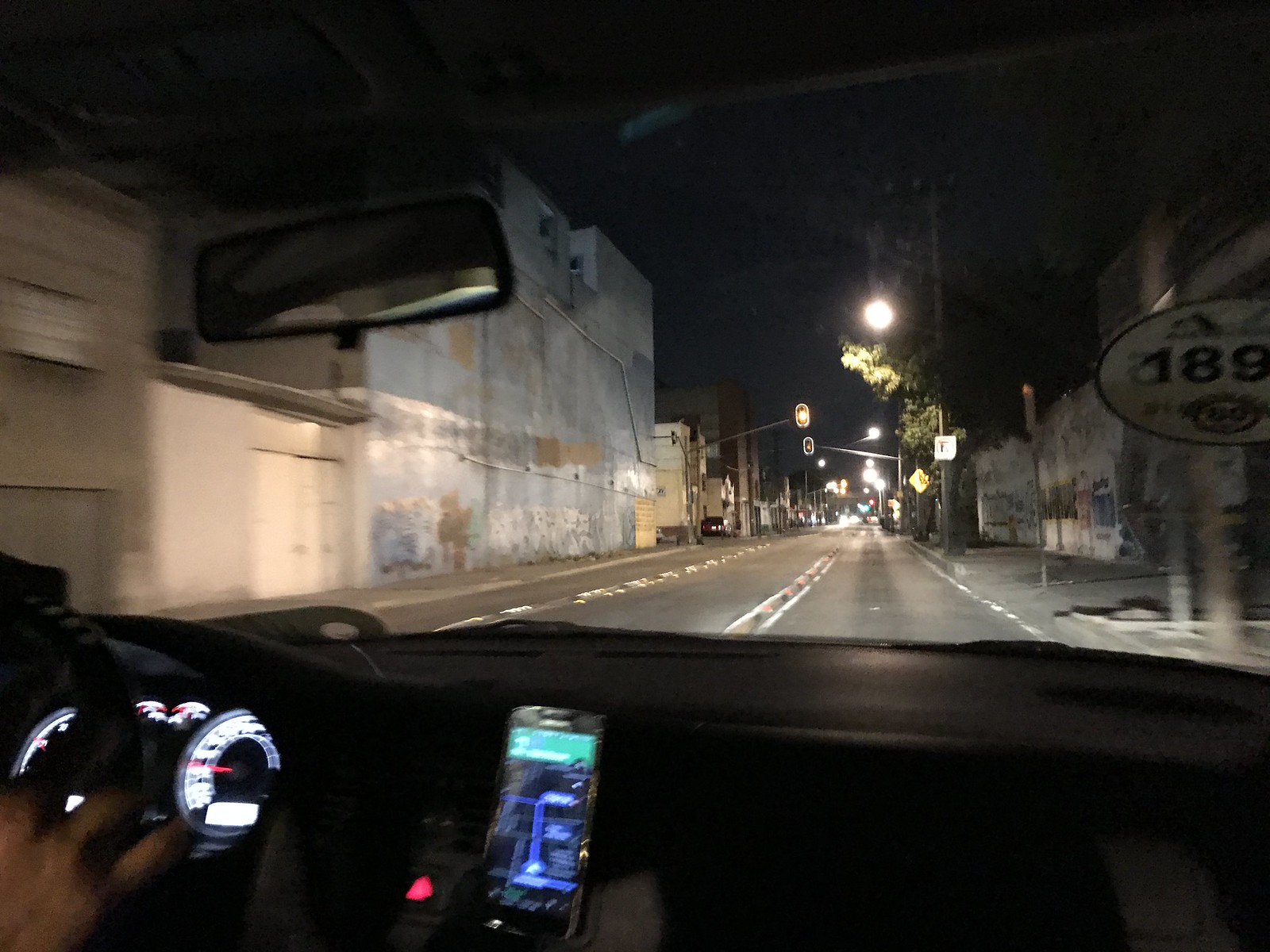The photograph captures an interior view from within a car during nighttime. The dimly lit interior reveals a blurry dashboard illuminated by various lights, indicating the vehicle's status. A driver's hand is firmly gripping the steering wheel, suggesting an active navigation. Mounted centrally on the dashboard is a smartphone displaying a navigation application, guiding the route ahead. Through the car's windshield, the scene transitions to an external view of a narrow street bathed in the soft glow of streetlights. Flanking the road are worn, cement buildings that exhibit signs of neglect and weathering, hinting at a rundown area perhaps struggling with economic hardships. The juxtaposition of the illuminated, tech-centric car interior against the gritty, dilapidated urban backdrop invites a contemplative reflection on contrasting environments.